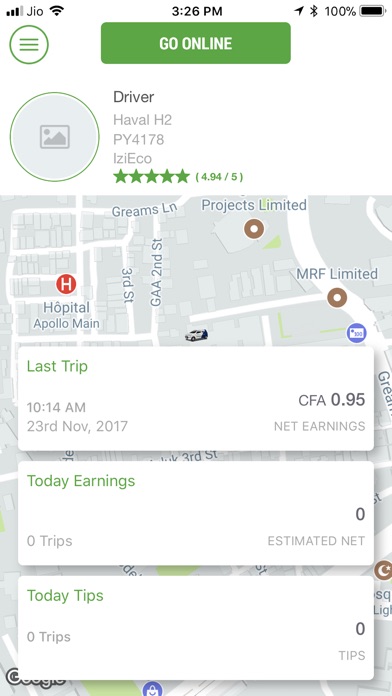The image resembles the interface of a popular mobile rideshare app, such as Uber or Lyft. At the center of the image is a detailed map displaying various recognizable locations, including a hospital, multiple buildings, and labeled street names. A car icon is prominently featured on the map, indicating the driver's position or activity.

Overlaid on the map are three distinct blocks of information. The top block, titled "Last Trip," shows financial details with "CFA 0.95" and "Net Earnings," though the specific earnings value is not provided. The middle block indicates the driver's activities for the day with sections labeled "Today's Earnings," showing an estimated net of zero and zero trips taken. The bottom block, "Today's Tips," also reflects zero trips and zero tips, suggesting the driver has not yet completed any rides for the day.

Additionally, the profile information for the driver is detailed. The driver’s vehicle is a Haval H2 with the license plate PY4178, and the driver’s name or identifier is Izzy Eco. The driver boasts an impressive rating of 4.94 out of 5 stars, signifying a high level of customer satisfaction.